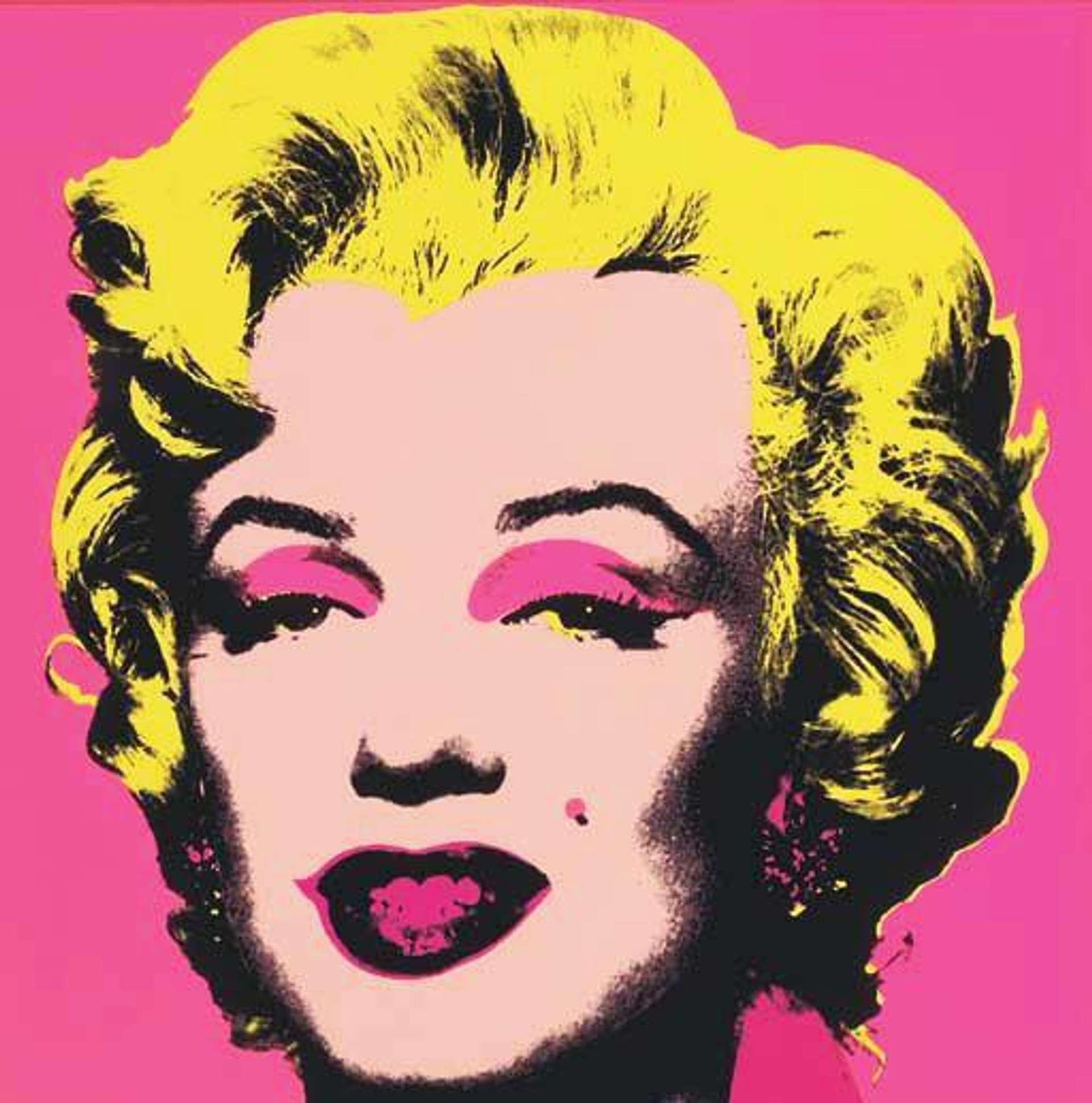This artwork is a vibrant digital illustration of Marilyn Monroe, rendered in a neon-infused style reminiscent of Andy Warhol's iconic pop art. Marilyn's hair is a striking, unnatural yellow with deep black accents to delineate the outlines and shadows. Her skin is a light pink, harmonizing with the bold pink background. Her makeup stands out with neon pink eyeshadow and eyeliner, and her lips are similarly vivid, matching her eye makeup. Her trademark mole is subtly tinted pink. The portrait mainly focuses on Marilyn's head, with her neck and chin area portrayed in black shadow, adding depth and texture. The combination of these elements creates a mesmerizing, colorful homage to Marilyn Monroe, showcasing the hallmark features of Warhol’s celebrated artistic style.